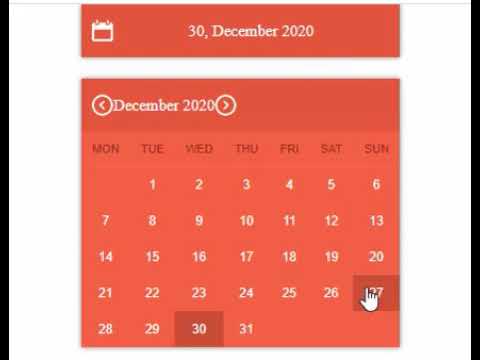The image showcases a digital calendar displayed on what seems to be a cell phone screenshot, largely dominated by a red theme. The top part of the calendar prominently displays the date "30th December 2020," indicating it is from the year 2020. The entire calendar interface, from the header to the individual dates, is rendered in varying shades of red, possibly invoking a festive connection to the month of December. However, there are no identifying company logos, dismissing the possibility of it being directly related to a specific corporation like Target, despite the similar color scheme.

Below the main date header, the calendar for the month of December is presented in a grid format. On the top left corner of this grid, a small arrow icon indicates the ability to navigate back to previous months, while a corresponding arrow on the top right corner suggests moving forward to months in the year 2021. Each date within the grid is numerically indicated in a lighter shade of red, differentiating it from the bold top header. Additionally, the image captures a moment where a finger appears poised to select the date "27th December," highlighting an interactive element of the digital calendar interface.